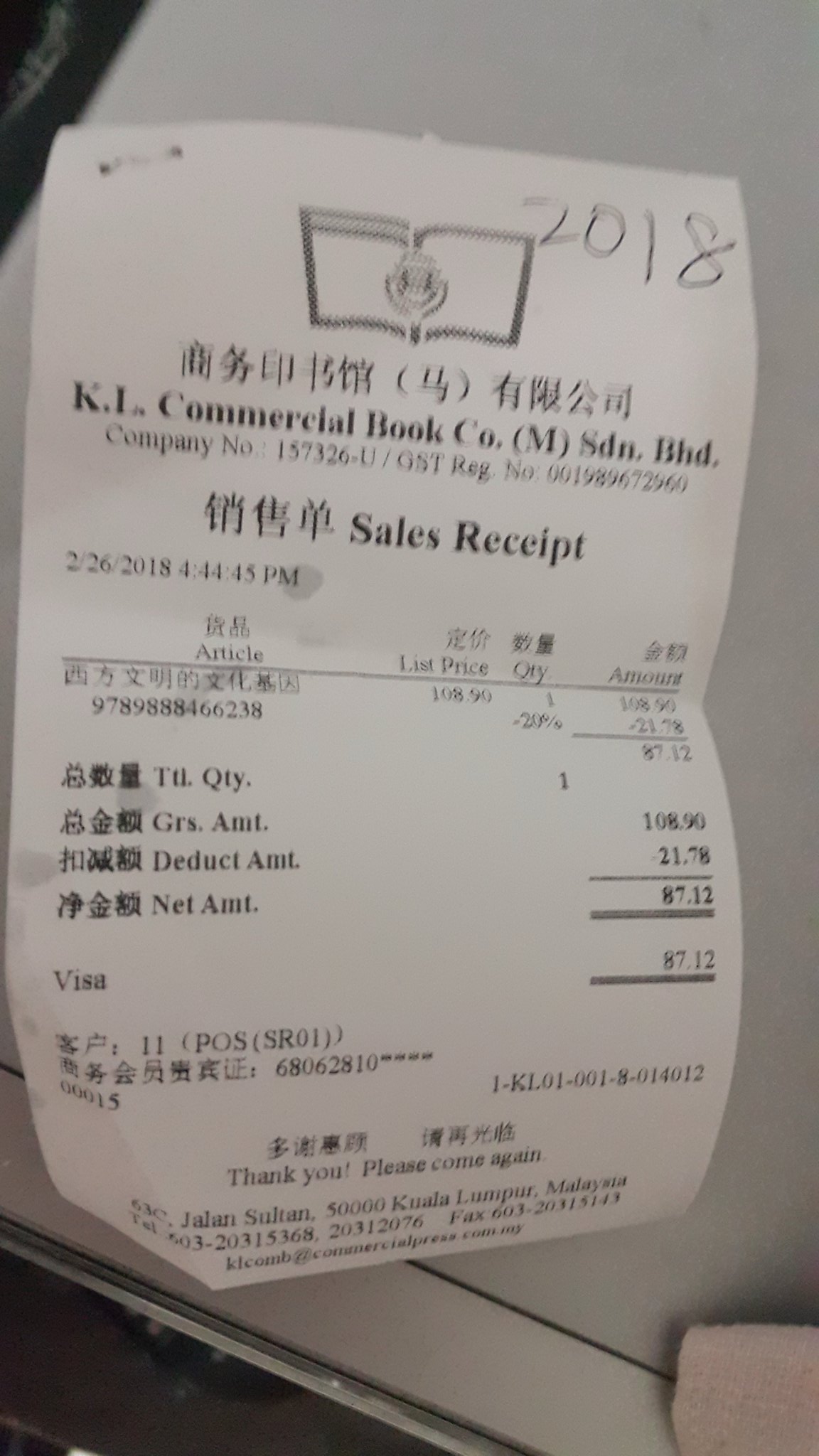This image captures a close-up view of a receipt. The receipt is white with black text and appears to have been photographed indoors. Notably, the upper right corner of the receipt bears the handwritten year "2018." The receipt's header reads "KI Commercial Book Company SDN.BHD," followed by their company number "157326-U" and GST registered number "001-989-672-960." The receipt is labeled as a "Sales Receipt" and is dated February 26, 2018, at 4:44 p.m.

The purchase details include an item with the identifier "978-988-846-662-38," originally priced at $108.90, but listed with a 20% discount, reducing the price to $87.12. The total amount charged was paid using a Visa card. At the bottom of the receipt, there is a courteous note stating, "Thank you, please come again," along with the address "Jalan Sultan, 50000 Kuala Lumpur, Malaysia." Additional contact information, including phone and fax numbers, is also printed at the bottom.